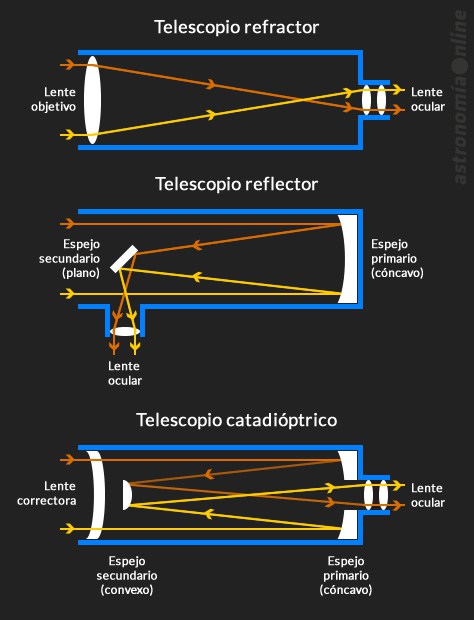The infographic, entirely in Spanish, illustrates the internal workings of three types of telescopes: refractor, reflector, and catadioptric, against a black background with white sans serif text. At the top, labeled "Telescopio Refractor," a rectangular diagram features a white oval on the left marked "Lente Objetivo" and two smaller ovals on the right labeled "Lente Ocular." Orange and yellow lines, representing light paths, crisscross through these ovals. Below, a second labeled "Telescopio Reflector" shows an open-ended rectangle starting with "Espejo Secundario Plano" (secondary flat mirror) and lines indicating light reflection towards "Espejo Primario Cóncavo" (primary concave mirror). The final diagram, labeled "Telescopio Catadioptrico," details a more complex layout featuring "Lente Correctora" (corrective lens) at the left and mirrors "Espejo Secundario Convexo" (secondary convex mirror) and "Espejo Primario Cóncavo" (primary concave mirror) directing light to "Lente Ocular." The consistent use of color-coded lines and detailed components across all three images effectively explains the different pathways light takes within each telescope type.